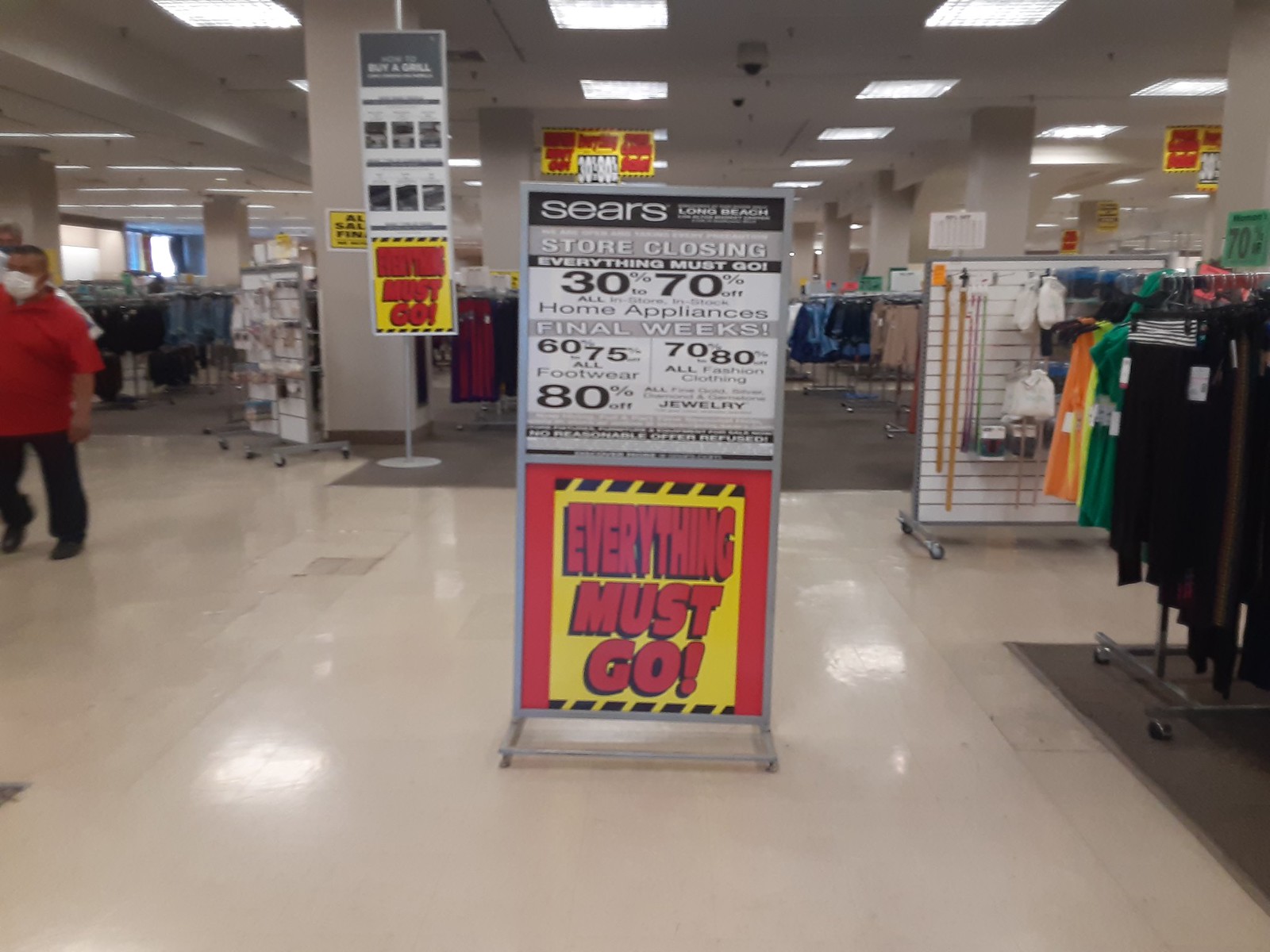The photograph depicts the interior of a Sears department store that is in the process of closing down. The image, slightly wider than tall, shows a prominent sign in the center of the walkway. The sign has a black bar at the top with small, white text that reads "Sears Long Beach." Below this, larger red text on a yellow background announces "Store Closing, Everything Must Go, 30% to 70% Off Home Appliances, Final Weeks," with additional discounts for specific categories such as "60-70% Off All Footwear" and "70-80% Off All Fashion Clothing." A red message on a yellow background at the bottom reiterates "Everything Must Go." On the left side of the image, a person wearing a red polo shirt, black pants, and a white face mask can be seen. To the right, racks of clothing and accessories, including shirts and belts, are displayed. The store has a tiled ceiling with square lights, and additional sales signs hang from the ceiling throughout the background.